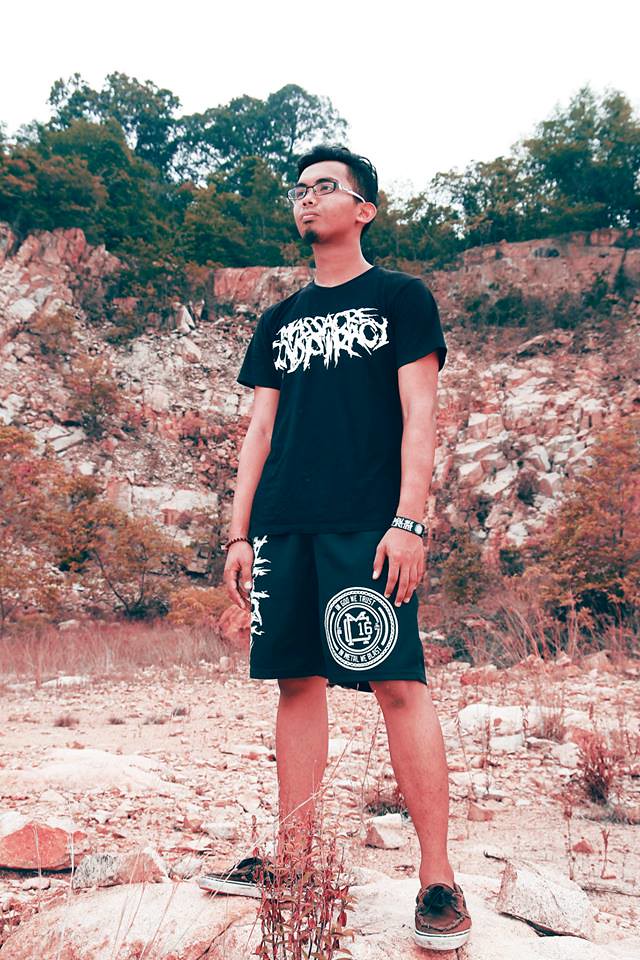In the image, a young man is standing confidently on a rock in a natural, rocky, and hilly landscape. The terrain, surrounding him, consists of similar rocks with patches of plants and scrub brush, leading up to a green canopy of trees at the top. The sky above appears white, creating a serene backdrop. 

The man is dressed in a coordinated black outfit, featuring black shorts adorned with white designs and possibly a round symbol on the left leg. His black t-shirt has white text in an illegible font. He is sporting black tennis shoes with hints of brown. His accessories include a wristband on his left arm and a bracelet on his right arm. He has short, dark black hair, a small goatee, and is wearing rectangular glasses. 

His stance on the rock and distant gaze suggest he is posing intentionally for the camera, capturing a moment of tranquility far removed from civilization.